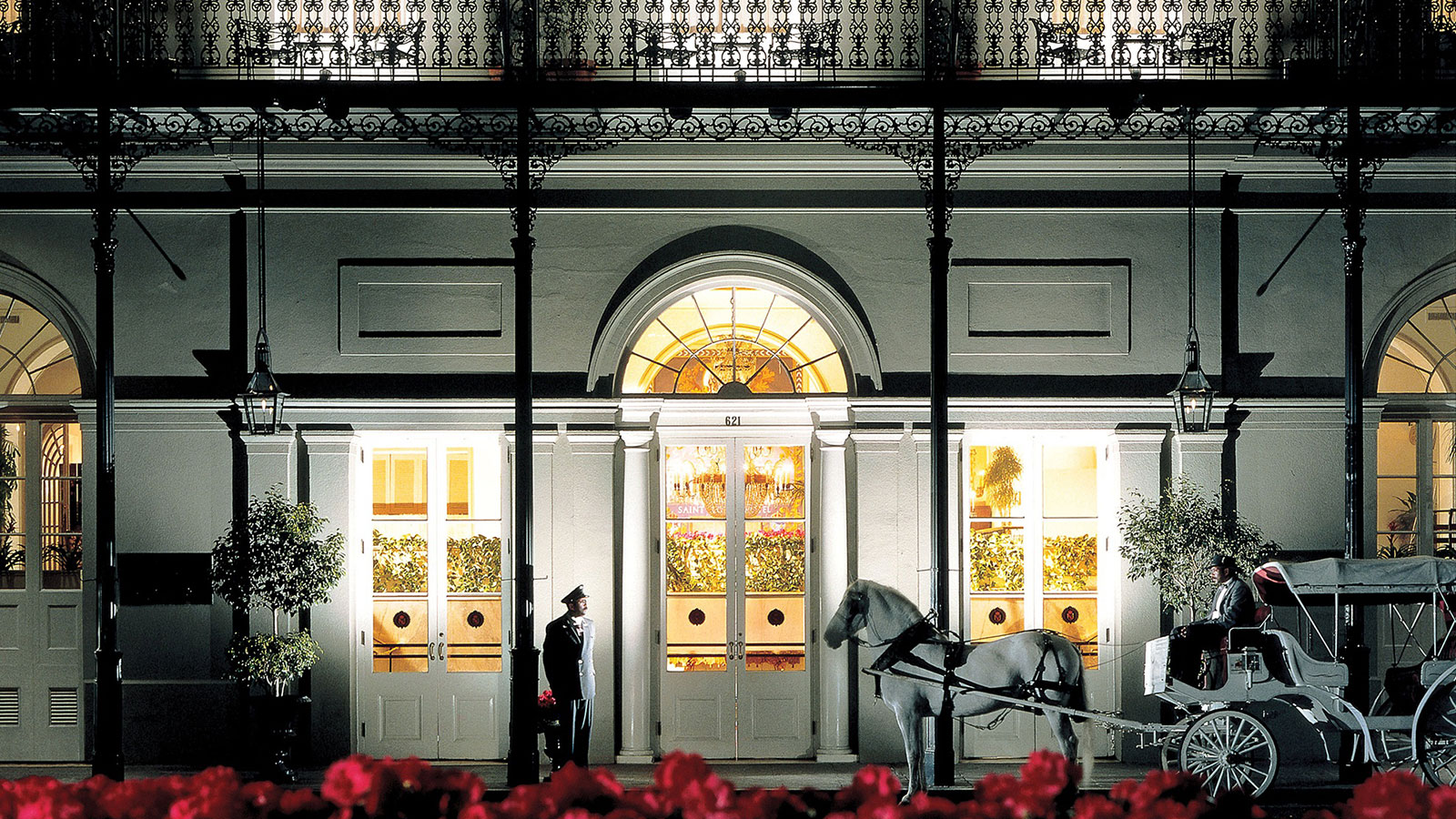The image depicts a large, elegant white building with black wrought iron detailing. The structure features three glass-paneled doors, with a central door surmounted by an arched window. Several additional windows are visible, indicating that the building is quite expansive. In front of the building, there is a distinguished man in a black suit and hat, resembling an attendant or doorman, standing with his hands behind his back. To the right of the man is a white horse-drawn carriage, attended by a carriage driver, and harnessed to two horses. The carriage is parked directly in front of the building. Bright red flowers line the bottom foreground of the image, and there is a green tree to the left. Despite the nighttime setting, the building's interior is illuminated, casting a warm glow outside. The black wrought iron railing and swirly pattern details add a touch of sophistication to the scene.